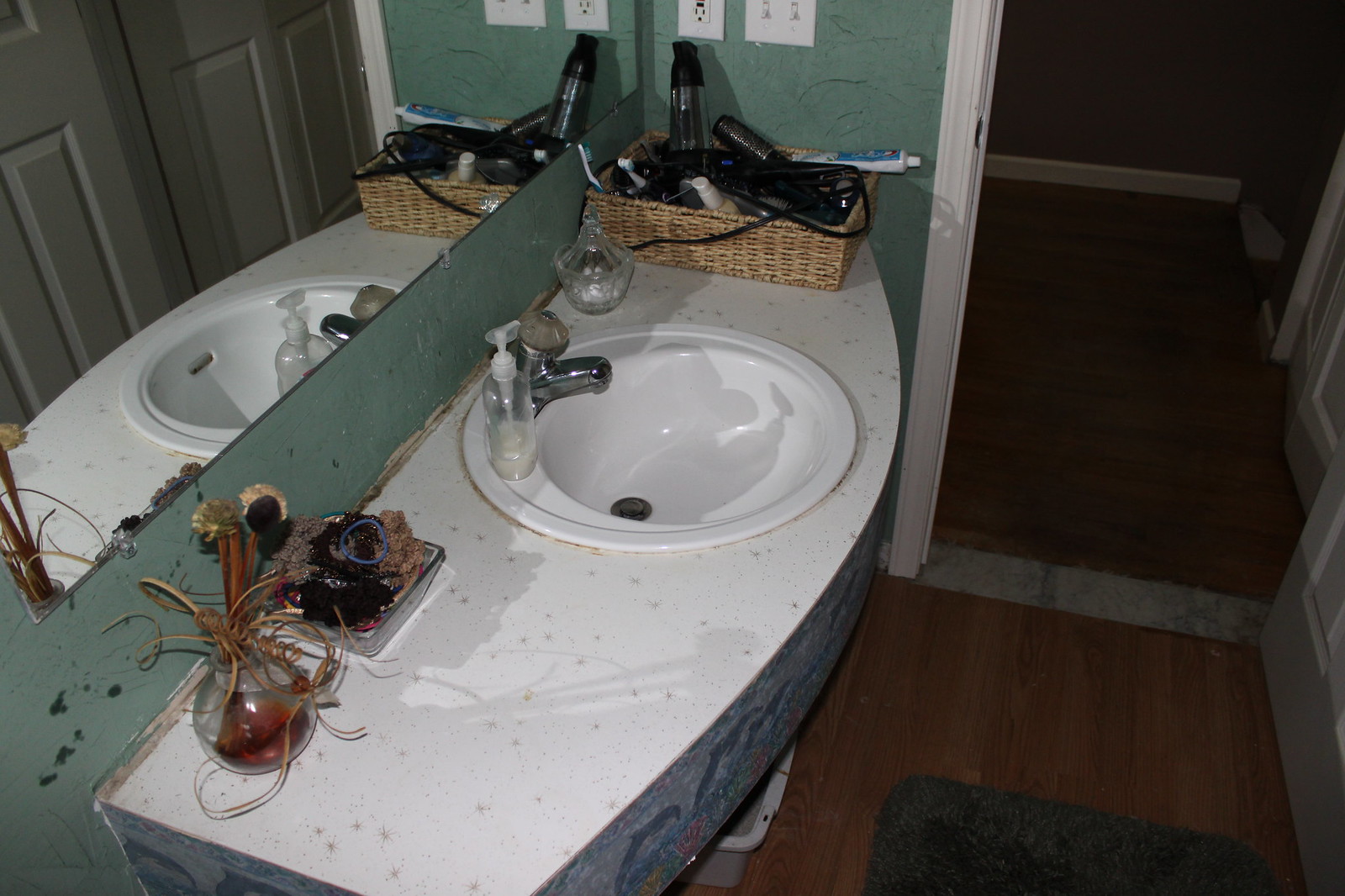The image depicts an older-style bathroom vanity viewed from a higher angle. The floor appears to be brown, likely a faux wood material rather than real wood. The vanity itself is bluish in color, featuring a laminate surface. However, the caulking around the vanity's edge is visibly dirty and aged. The wall behind the vanity is painted a different shade of blue, with noticeable paint chipping in some areas. The sink is circular, with similar brownish, mildewy caulking around its edge, and is equipped with a silver-tone faucet. On the vanity, there is a white soap pump and a glass container with a lid. To the right, a light tan rectangular basket holds various appliances such as a hair straightener and hair dryer. On the left side, there's an open container filled with items like scrunchies and a hair tie. Further left, a vase with dried, curling flowers adds a decorative yet weathered touch to the setting.